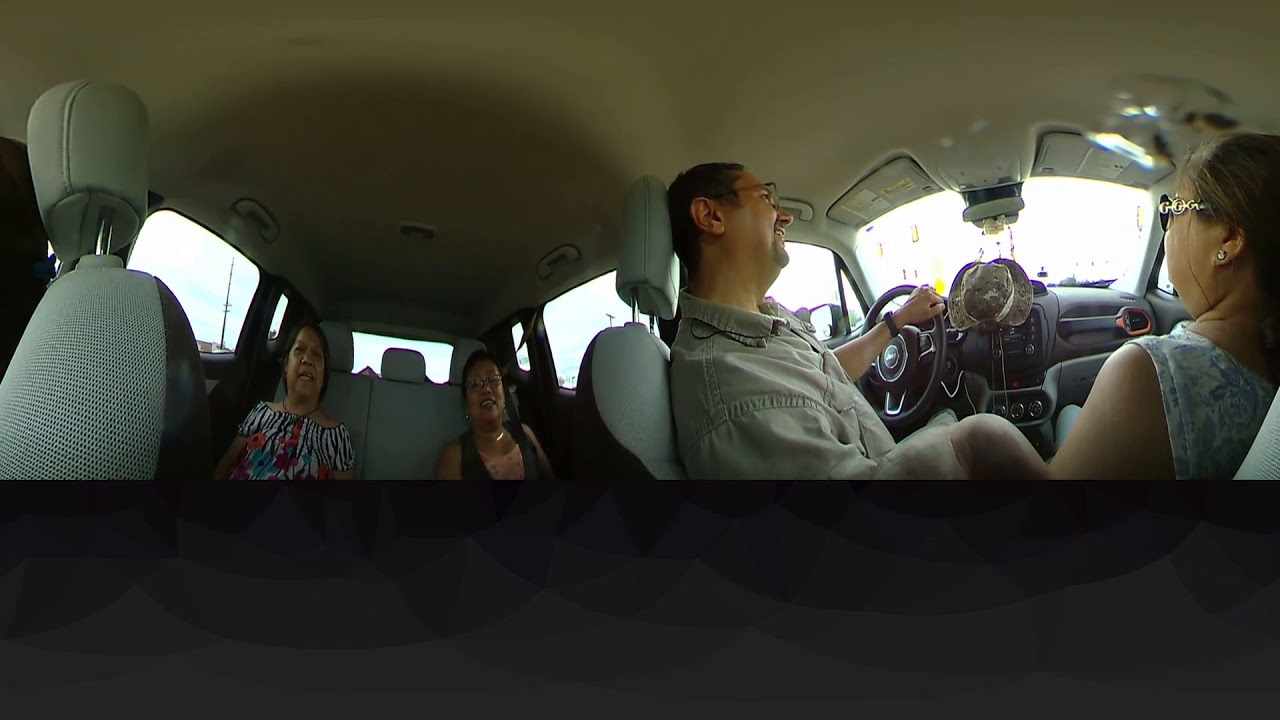This color photograph, in landscape orientation with a black strip across the bottom third, appears to be two combined images showing different parts of the same car. The right side features the front seat where the driver, a Southeast Asian man in his 50s with dark hair, glasses, a tan shirt, and a little facial hair, is seen from the side. He is smiling and has his left hand on the steering wheel. His sunny surroundings are visible through the windshield, along with a chain and a hat hanging from the rear-view mirror. Beside him is a Southeast Asian woman, also in her 50s, wearing a sleeveless top, sunglasses, and an earring in her left ear. Her hair is pulled back and she is looking out the windshield.

On the left side of the image, the backseat is depicted, showing two women, likely of Southeast Asian descent and in their 50s. Both women, facing the viewer and appearing to talk, have dark hair and features. The woman on the left wears a floral black, white, and blue top, while the woman on the right sports a low V-cut black top and a gold necklace. The car has a tan-colored interior, and the scene is bright, suggesting daytime.